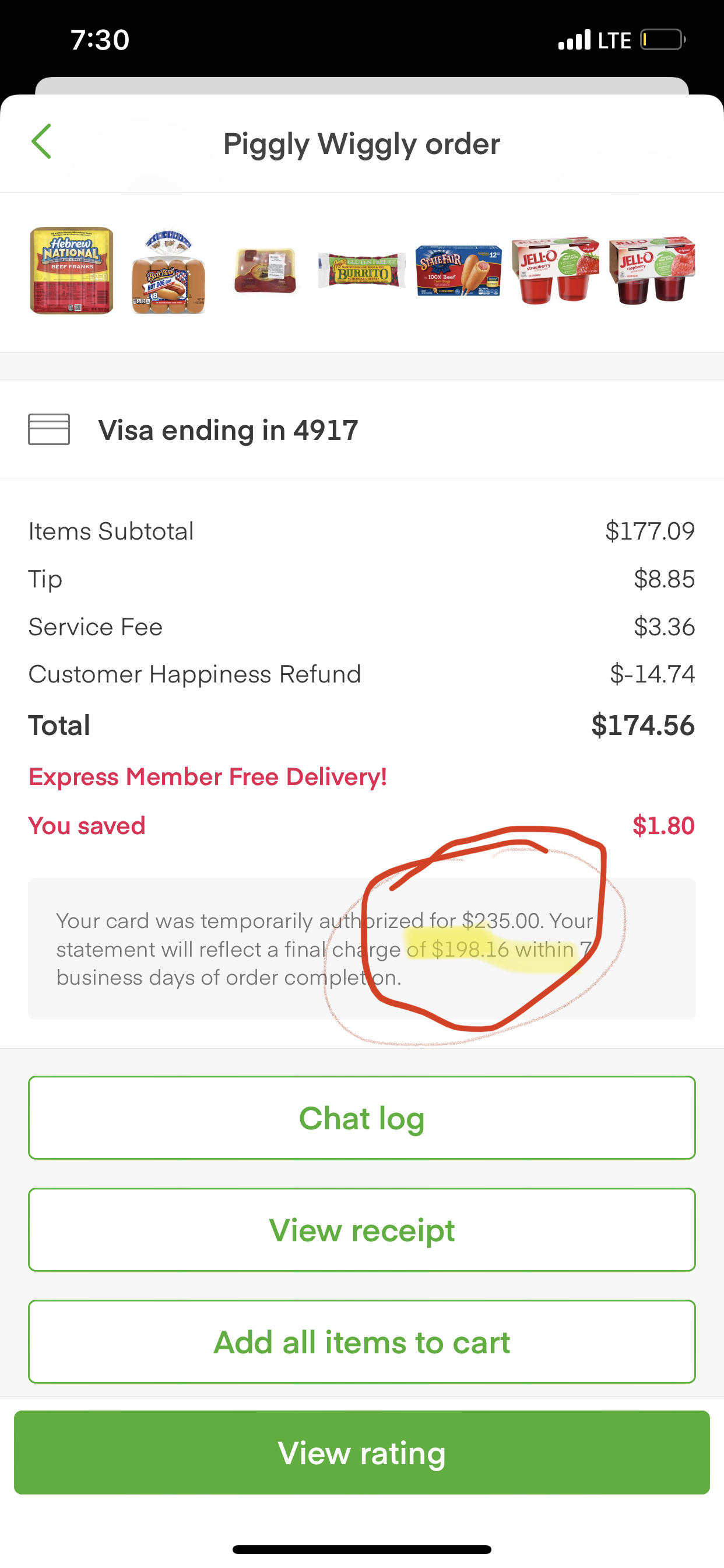A screenshot captures someone's Instacart order on their mobile phone, taken at 7:30. The phone's battery is critically low. The order is from Piggly Wiggly and comprises seven items, including Jell-O, bread, and popsicles, although some other items are difficult to discern. The payment method shows a Visa card ending in 4917. The item subtotal amounts to $177.09, with an added tip of $8.85, a service fee of $3.36, and a customer happiness refund of -$14.74, bringing the total to $174.56. The user saved $1.80 as an Express member, and the highlighted billing note indicates that the card was temporarily authorized for $235.00, with a final charge of $198.16 to reflect on the statement within seven days. The overall expense is considerable.